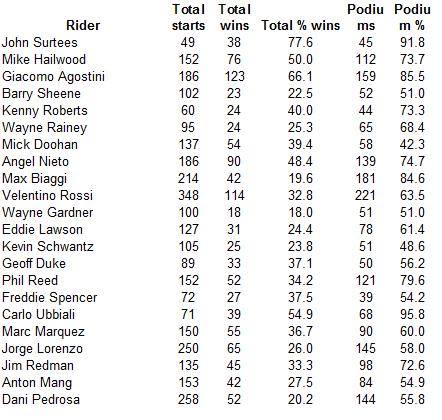The image is a black-and-white data table, featuring black text on a white background. The table includes six columns labeled "Writer," "Total Starts," "Total Wins," "Total Percentage of Wins," "Podiums," and "Podium Percentage." The "Writer" column lists approximately 30 to 40 names of notable individuals, including John Surtees, Mike Hailwood, Giacomo Agostini, Barry Sheene, Kenny Roberts, Wayne Rainey, Mick Doohan, Ángel Nieto, Max Biaggi, Valentino Rossi, Wayne Gardner, Eddie Lawson, Kevin Schwantz, Geoff Duke, Phil Read, Freddie Spencer, Carlo Ubbiali, Marc Márquez, Jorge Lorenzo, Jim Redman, Anton Mang, and Dani Pedrosa. The remaining columns display various statistical data related to these individuals' achievements, such as the number of starts, wins, win percentages, podiums, and podium percentages. The data is presented in a straightforward manner without any images or additional graphics.